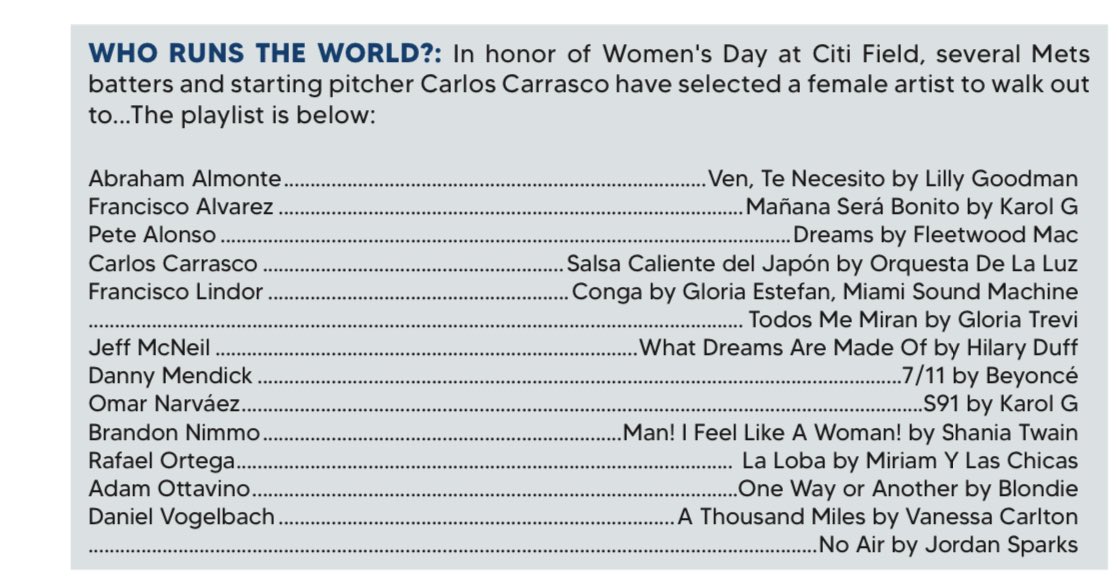This infographic titled "Who Runs the World" in navy blue celebrates Women's Day at Citi Field, showcasing several Mets batters and starting pitcher Carlos Carrasco, who have selected female artists for their walk-up songs. The pale gray background features black and navy blue text, listing players and their chosen songs. The playlist includes: 

- Abraham Almonte: "Ven, Te Necesito" by Lily Goodman
- Francisco Alvarez: "Mañana Será Bonito" by Carol G
- Pete Alonso: "Dreams" by Fleetwood Mac
- Carlos Carrasco: "Salsa Caliente del Japón" by Orquesta de la Luz
- Francisco Lindor: "Conga" by Gloria Estefan and Miami Sound Machine, and "Todos Me Miran" by Gloria Trevi
- Jeff McNeil: "What Dreams Are Made Of" by Hilary Duff
- Danny Mendick: "7/11" by Beyoncé
- Omar Narvaez: "S91" by Carol G
- Brandon Nimmo: "Man! I Feel Like a Woman" by Shania Twain
- Rafael Ortega: "La Loba" by Miriam y Las Chicas
- Adam Ottavino: "One Way or Another" by Blondie
- Daniel Vogelbach: "A Thousand Miles" by Vanessa Carlton and "No Air" by Jordin Sparks

This detailed playlist highlights the players' tributes to female artists in honor of the occasion.